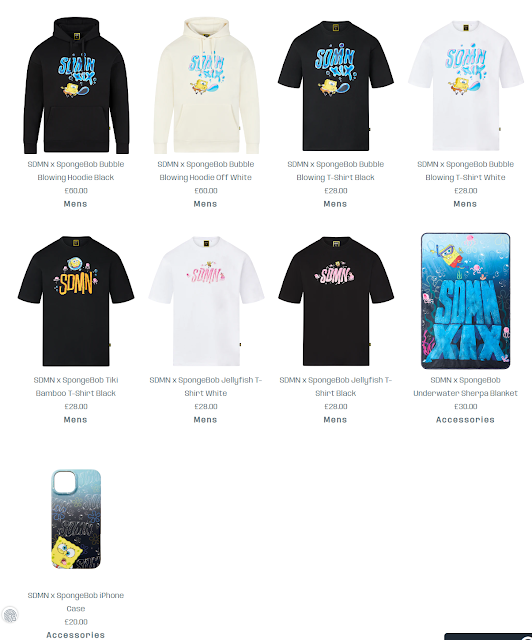The image displays a section of a website selling t-shirts and various other items. The layout consists of three rows; the first two rows each feature four items, while the last row has a single item.

In the first row, there are several products:
1. A black hoodie labeled as "SDMN x Spongebob Bubble Blowing Hoodie Black." The specifics of the price aren't clear due to low image resolution, but it is categorized under men's apparel. The hoodie features a design of Spongebob blowing a bubble.
2. An off-white hoodie described as "SDMN x Spongebob Bubble Blowing Hoodie Off-White," also for men. Again, the price is indiscernible.
3. A black short-sleeved t-shirt titled "SDMN x Spongebob Bubble Blowing T-Shirt Black," priced at 28 pounds and listed under men's apparel. This shirt displays the same Spongebob design.
4. A white short-sleeved t-shirt called "SDMN x Spongebob Bubble Blowing T-Shirt White," similarly priced at 28 pounds and for men. It also showcases the same bubble-blowing Spongebob graphic.

The image quality is quite pixelated, making some details and prices difficult to read. The recurring theme among these items is the collaboration between SDMN and Spongebob, featuring consistent graphic designs centered around Spongebob blowing a bubble.